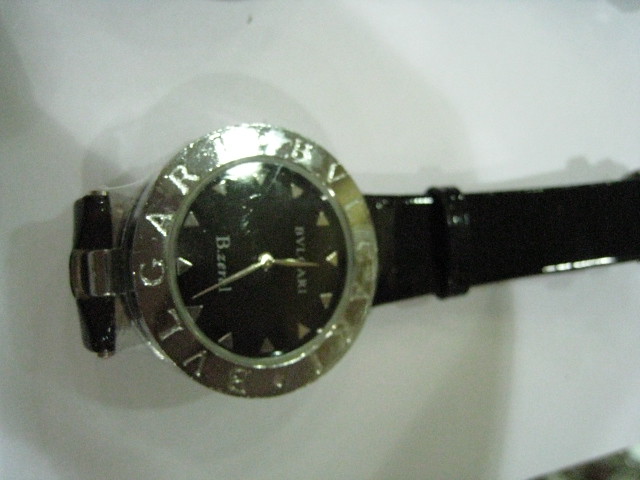This detailed photograph captures a stylish women's wristwatch from an aerial perspective. The watch is artfully placed on a white hard surface, casting soft gray shadows over the left two-thirds of the image. The sophisticated timepiece features a black leather band, folded behind the watch such that it spans diagonally from left to right. The round face of the watch is encircled with a sleek silver frame, while the interior boasts a black backdrop adorned with miniature silver triangle studs replacing numbers. In place of numerals, the perimeter of the face reads "BVLGAR" elegantly engraved in silver. Additionally, the watch has two shiny silver hands that indicate the time as 12:26. A subtle text, partially obscured by glare, appears above the 6, hinting at further branding or design details.